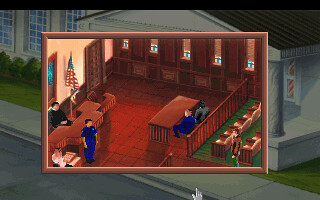The composite image showcases two perspectives of a courthouse. The background features the courthouse's exterior, revealing its architectural elements with a classic façade that includes columns, a visible roof, several windows, and the main entrance door. The monochromatic tones of gray and white accentuate the timeless design, though the actual courthouse is not explicitly identified. Dominating the central portion of the image is a prominent rectangular inset depicting the courthouse interior. The inside scene is rendered in warmer tones, with a brown floor and green jury area. Benches are arranged for the jury, and a lawyer is seen seated at a desk with a client, accompanied by another individual. A police officer stands attentively in front of the judge, who is positioned behind a bench adorned with an American flag. The juxtaposition effectively captures both the stately exterior and the detailed, procedural interior of the courthouse environment.